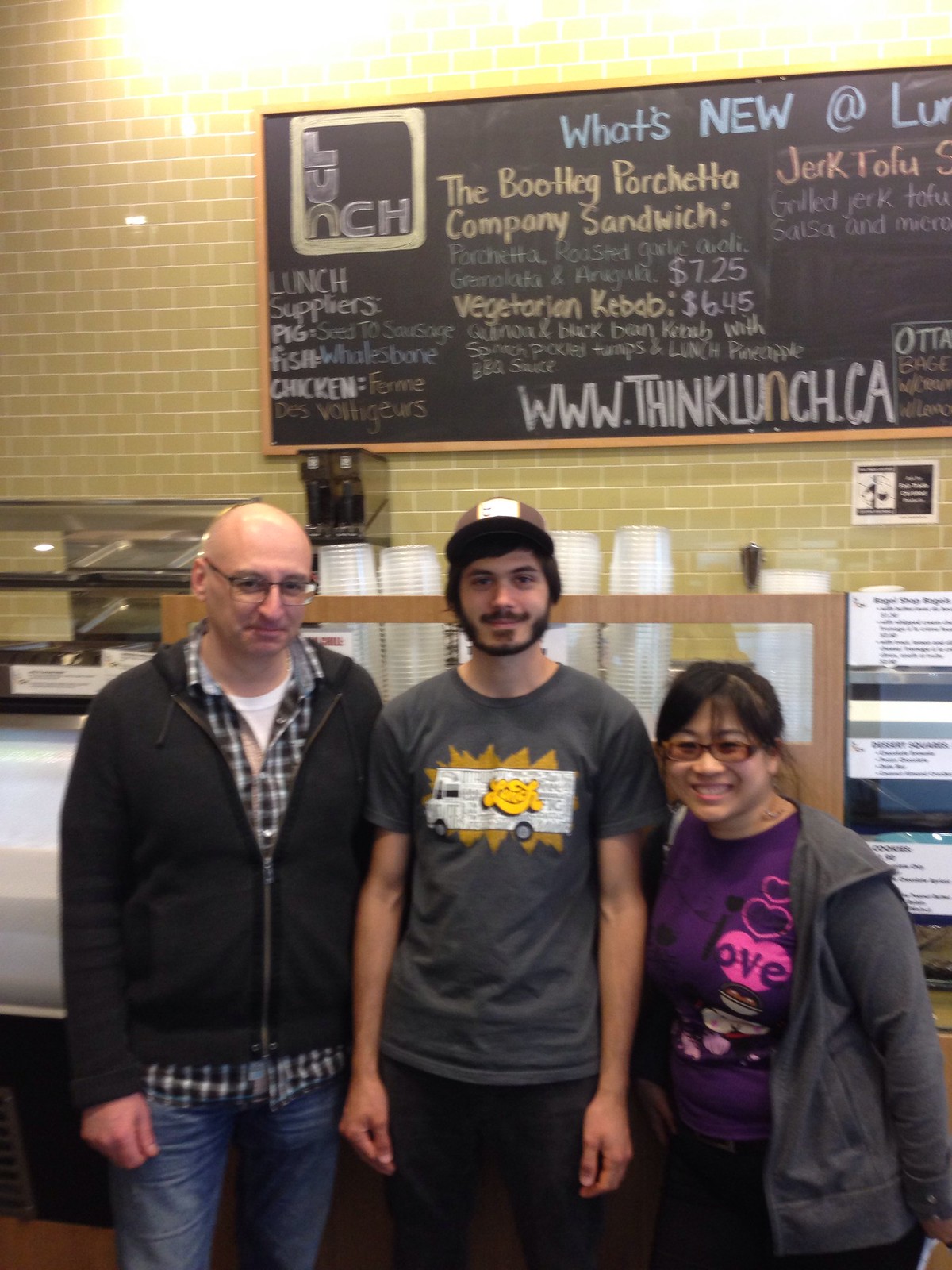In a brightly lit restaurant setting, three individuals pose beneath a meticulously detailed chalkboard menu. On the left stands a bald Caucasian man with glasses. He sports a black jacket, zipped halfway up, revealing a plaid black-and-white-striped shirt layered over a white T-shirt. He wears blue jeans, and his left hand hangs just past his hip. In the center is a man with black hair, a full beard, and a mustache. He wears a gray T-shirt adorned with an illustration of a white box truck and vivid orange accents, along with black pants and a brown hat featuring a white patch. On the right, the shortest of the trio is a woman with a warm, big smile. Her black hair is pulled back, and she dons tinted glasses. She is dressed in a purple shirt decorated with hearts, one of which features the letters "OVE," and a gray jacket over the top.

Behind them, a yellow brick wall supports a large black chalkboard brimming with colorful chalk inscriptions. At the top, bold white and blue chalk letters announce "What's New," followed by a highlighted yellow section listing "The Booty Porchetta Company Sandwich." In the upper left corner, a beige square vertically spells out "LUNCH" in fun lettering. Additional offerings and their prices are listed beneath, in various colored chalk, with the website "www.thinkluncheon.ca" inscribed at the bottom. Stacks of clear plastic containers are visible in the background, contributing to the bustling atmosphere of the eatery. A bright white light from the upper left casts a warm glow over the scene, completing the lively and inviting ambiance of this restaurant snapshot.